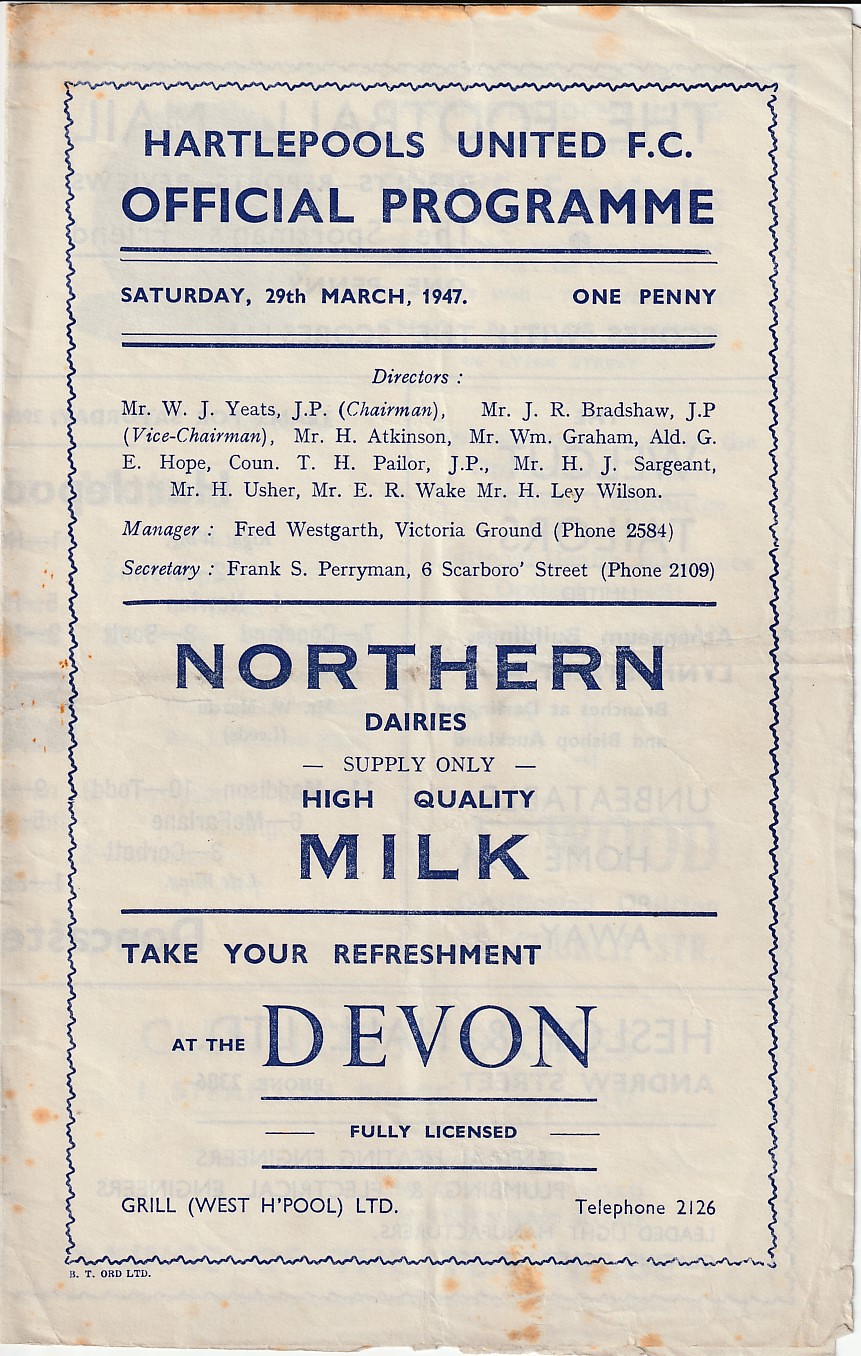The image displays an aged, slightly singed white paper, which appears to be Hartlepool United FC's official program from March 29th, 1947, priced at one penny. The paper is bordered and lettered in blue with a rusty orange patina indicating its age. The layout divides the content into three sections: the top third of the page bears the program's title and date, the middle third lists the directors, managers, and secretaries of the club, while the bottom third contains advertisements. The primary advertisement, placed centrally, is for Northern Dairies, which promotes high-quality milk. Another advertisement below it suggests patrons 'Take Your Refreshment at the Divan,' indicating it is fully licensed. The entire piece takes up the entirety of the image, providing a nostalgic glimpse into the history of a 1947 soccer match program.